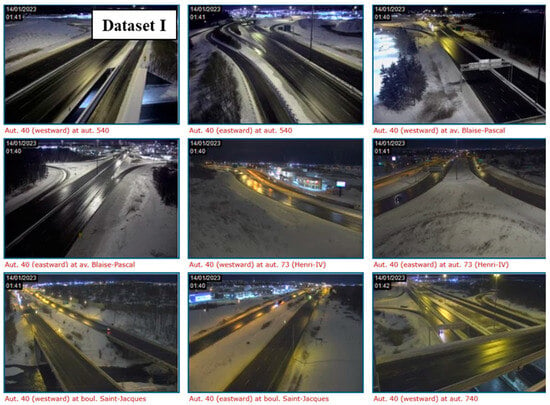The image features nine stills from security camera footage of different highways or roads at night, arranged in a 3x3 grid with a white border around each photo. Each photo has red letters underneath indicating the location and time. The top-left image, labeled "Data Set 1," shows a two-lane highway, one lane going in each direction, with a timestamp of 1:41 and snow-covered roads glistening from street lamps. The top row continues with similar scenes of snowy highways from different angles. The middle row's center image is taken from atop a hill, featuring roads with snow in the median and buildings lit up in the distance. The bottom row offers an aerial perspective of highways lined with snow and additional cameras set up over the roads, further emphasizing the surrounding illuminated businesses and cityscape. Each photo captures the serene, snowy night, reflecting the icy conditions of the roads.